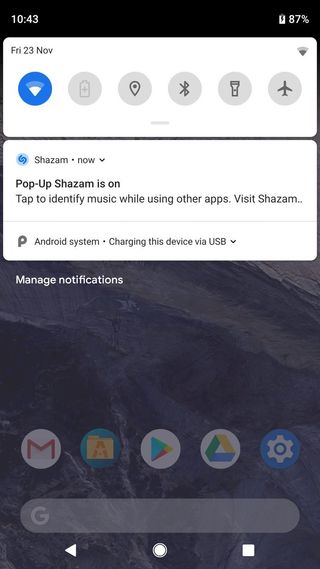A detailed smartphone screenshot exhibits the following elements:

1. **Status Bar**:
   - **Top Left Corner**: "10:43" time display, indicating AM or PM is not specified.
   - **Battery Life**: At 87% with a nearly full white battery icon against a black background.

2. **Notification Bar**:
   - **Date Information**: Situated in the upper left corner is a white rectangular bubble with rounded corners displaying "FRI 23 NOV" in gray.
   - **Icons**: Below the date bubble:
     - A blue circle featuring an upside-down triangle with a light blue top and white tip.
     - Series of gray circles with various symbols:
       - First Gray Circle: Faint outline of a gray battery.
       - Second Gray Circle: Teardrop-shaped icon with a black border and central dot.
       - Third Gray Circle: "X" with black triangles on top and bottom.
       - Fourth Gray Circle: Flashlight icon.
       - Fifth Gray Circle: Black airplane indicator.

3. **Notifications & System Information**:
   - **Left Section**: 
     - Blue emblem with two dark blue "C" shapes intertwined.
     - "SH.S" (suspected partial "Shazam" text) followed by "NOW", an arrow pointing down, and "POP-UP SHAZAM."
     - Guidance to tap 'T' to identify music while using other apps, along with "Visit Shazam...", with "VS." in capital letters.
   - **Below First Section**: 
     - Large gray 'P' indicating Android system notification.
     - "Charging this device via USB" with "Charging" and "USB" capitalized with a black downward arrow.

4. **Bottom Icons**:
   - Five circular app icons:
     - Red "M" on a white background.
     - Yellow envelope on a blue background.
     - Blue arrow with a red and yellow line, pointing right on a white background.
     - Familiar recycling symbol with green, yellow, and blue colors, next to a white sprocket inside a blue circle.
     - "G" representing Google text, light in color on a grayish bubble.

5. **Action Icons**:
   - Bottom section features navigational icons:
     - A left-pointing white arrow within a black circle.
     - Central square icon in white representing an apparent home or app switch button.

6. **Background**: The background is largely black, providing high contrast for white texts and icons, enhancing readability.

This screenshot intricately details a smartphone's screen capturing the status bar, notifications, and navigational icons providing insights into the device state and usage.